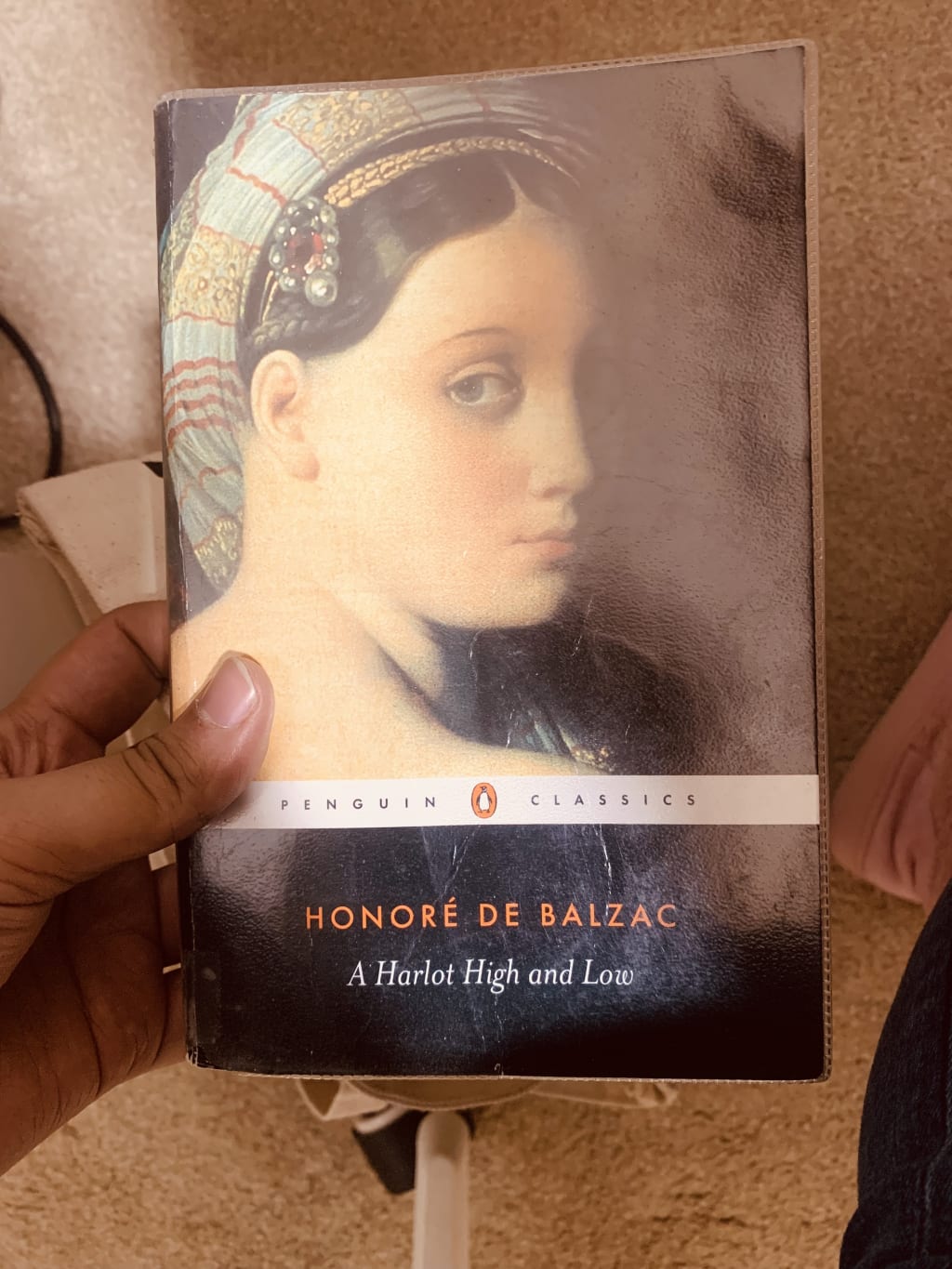In the image, a close-up photograph showcases a person holding a book titled "Honoré de Balzac: A Harlot High and Low," published by Penguin Classics. The individual’s dark-skinned hand is visible, with the thumb and fingers grasping the left side of the book, while part of their feet and a piece of jeans are discernible to the right. The cover art features a pale-skinned woman in Renaissance-style attire, looking over her right shoulder with a subtle, contemplative expression. She wears a multifaceted headdress combining light blue, yellow, and red tapestry elements, adorned with a prominent brooch and a pearl trinket. This headpiece drapes elegantly down her back. The background reveals a room with warm, beige carpet and pink walls, adding a domestic ambiance to the scene.